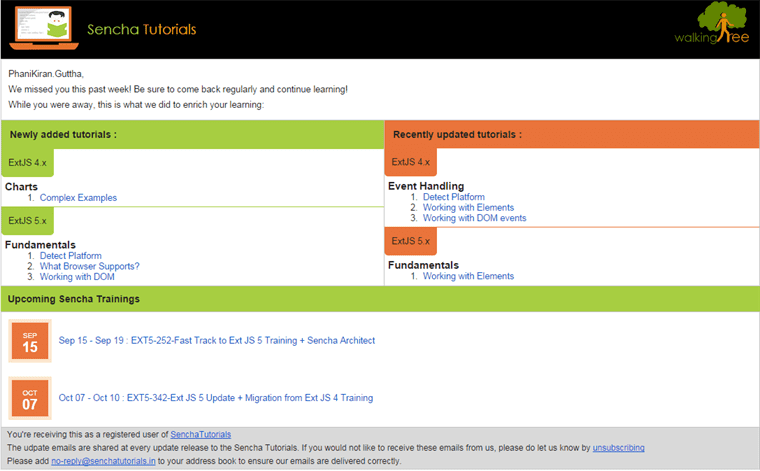**Detailed Image Caption:**

The image showcases a screenshot of a website with various sections dedicated to tutorials and upcoming training sessions. 

**Top Section:**
- **Title Bar:** A black title bar spans the top of the page. On the left, "Sencha" is written in green text, and "Tutorials" in orange text. An icon featuring an orange laptop with a person depicted inside it appears to the left of this text. On the far right, the logo displays an orange man standing in front of a green tree (without the trunk). Below the logo, the text reads "Walking" in green and "REE" in orange, with the orange man situated between these words.

**Middle Section:**
- **Message Block:** 
  - The background is white with small black text stating, "Panikiran Guta."
  - Below, there is a message reading, "We missed you this past week. Be sure to come back regularly and continue learning."
  - Another line follows: "While you were away, this is what we did to enrich your learning."

- **Tutorial Sections:**
  - **Newly Added Tutorials:** 
    - This section is marked with a green bar that stretches from the left to the middle of the screen, with bold black text stating, "Newly Added Tutorials, Ext.js 4.x."
    - Underneath, "Charts 1 Complex Examples" is written in blue text.
    - A green divider line shows the text "Ext.js 5.x and Fundamentals."
    - Below on a white background:
      1. Detect Platform
      2. What Browser Supports
      3. What is Working with DOM

  - **Recently Updated Tutorials:** 
    - This section mirrors the previous one but features orange colors and a similar layout.
    - The title "Recently Updated Tutorials, Ext.js 4.x" appears.
    - The blue text title reads, "Event Handling."
    - Below, the white background lists:
      1. Detect Platform
      2. Working with Elements
      3. Working with DOM Events
    - An orange divider line with black text contains "Ext.js 5.x," and underneath it, "Fundamentals" is written in blue text, followed by "Working with Elements."

**Bottom Section:**
- **Upcoming Sentient Trainings:**
  - A full-width green bar contains black text stating, "Upcoming Sentient Trainings."
  - Below, on the top left relative to the green bar, an orange box with white text reads "SEP 15," while blue text beside it reads, "SEP 15 to SEP 19, Ext. 5.x 252 Fast Track to Ext.js 5.x Training plus Sentient Architect."
  - Another similar setup below reads, "Oct 7" in white text within an orange box, and beside it in blue text, "Oct 7 to Oct 10, Ext. 5.x 342 Ext.js 5.x Update plus Migration from Ext.js 4.x Training."

**Footer:**
- A gray background bar at the bottom of the image reads, "You're Receiving This as a Registered User of Sentient Tutorials. The underpaid emails are shared at every update release to the SEP tutorials. If you would like to receive these emails from us, please do let us know by unsubscribing. Please add no-reply at sentienttutorials.in to your address book to ensure the emails are delivered correctly."